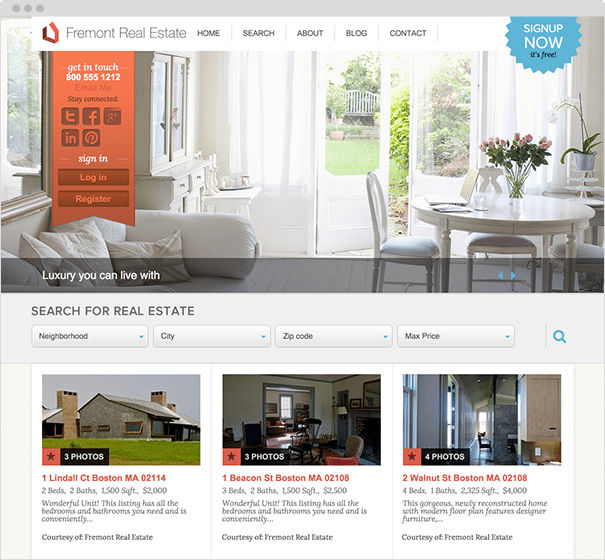Screenshot of a Fremont Real Estate website, viewed on an Apple iOS device, likely using a Mac browser. The web page features a sleek interface with a top left navigation bar containing options such as Home, Search, About, Blog, and Contact. To the right, a call-to-action banner invites users to "Sign Up Now - It's Free" with a ribbon icon next to it. Below this, a section prompting visitors to "Get in Touch" includes a phone number (800-555-1212) and an "Email Me" button. 

Further down, visitors can "Stay Connected" through various social media icons, including Pinterest, Indeed, Google+, Facebook, and possibly Tumblr. The page also offers Login and Register buttons for user access. All these elements are overlaid on a background image of a pristine, modern living room with white furniture, a dining table, and an open door revealing a lush, green backyard.

At the bottom of the page, there are three property listings with images and details. The first listing is for a house at First Lyndall Court, Boston, Massachusetts. The second, in the middle, is at First Deacon Street, Boston, Massachusetts. The third listing is located at Second Walnut Street, Boston, Massachusetts. Each property includes three to four photos, descriptions, and essential information such as the number of bedrooms, bathrooms, square footage, and price.